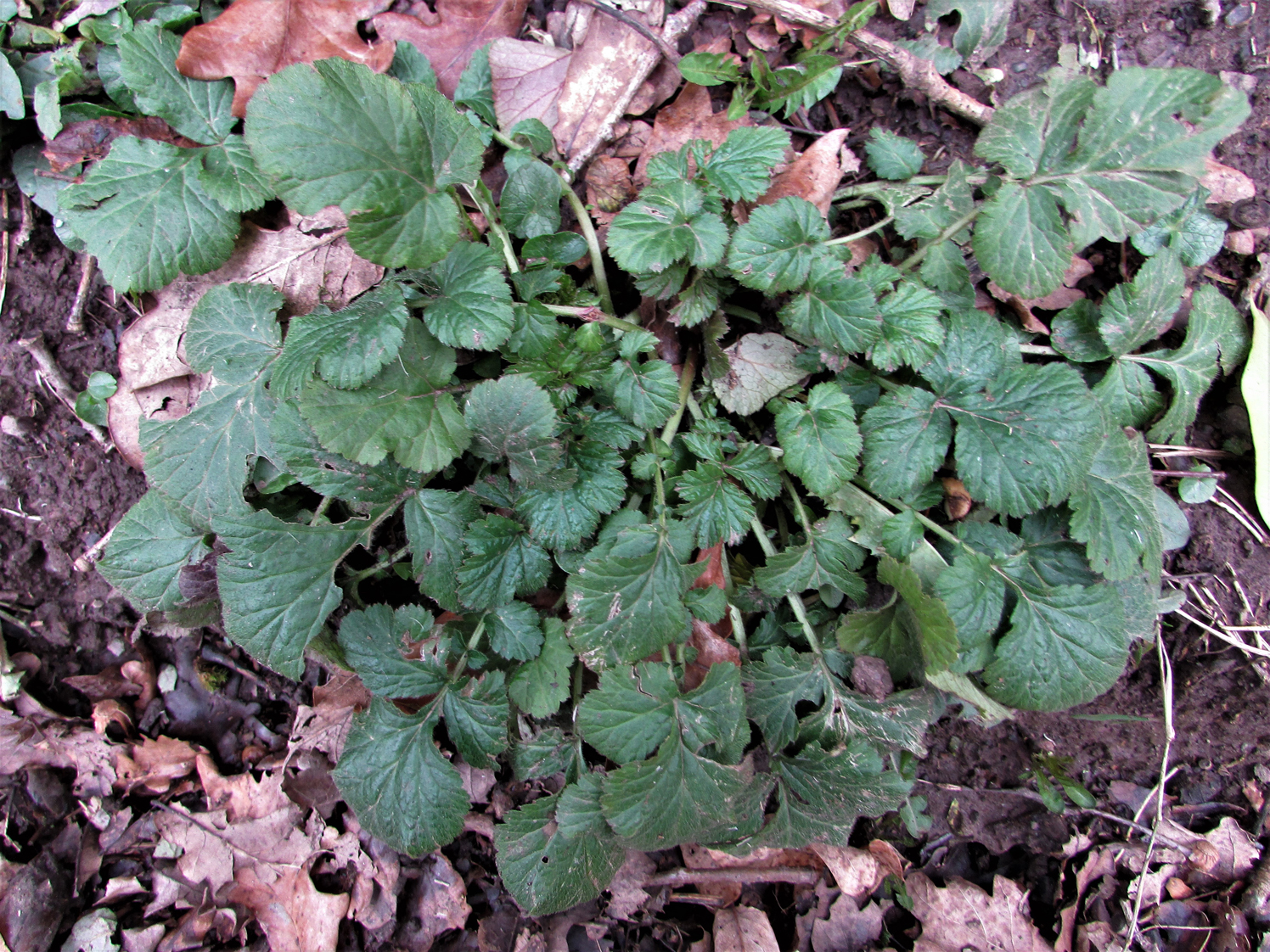This daytime outdoor photograph captures a close-up view of the ground, focusing particularly on a patch of weeds amidst a richly detailed scene. The image is taken from above, showcasing the moist, dark dirt around the edges. Interspersed throughout the dirt are various dead leaves in shades of brown, rust, tan, and gray, as well as old twigs. The central focus of the image is a collection of vibrant green weeds sprouting up, featuring heart-shaped leaves on sturdy green stems. These lush new plants are prominently positioned in the center, while more green leaves extend towards the upper left, disappearing out of the frame. The photograph beautifully contrasts the new growth with the remnants of past vegetation, highlighting a natural progression in the plant life.